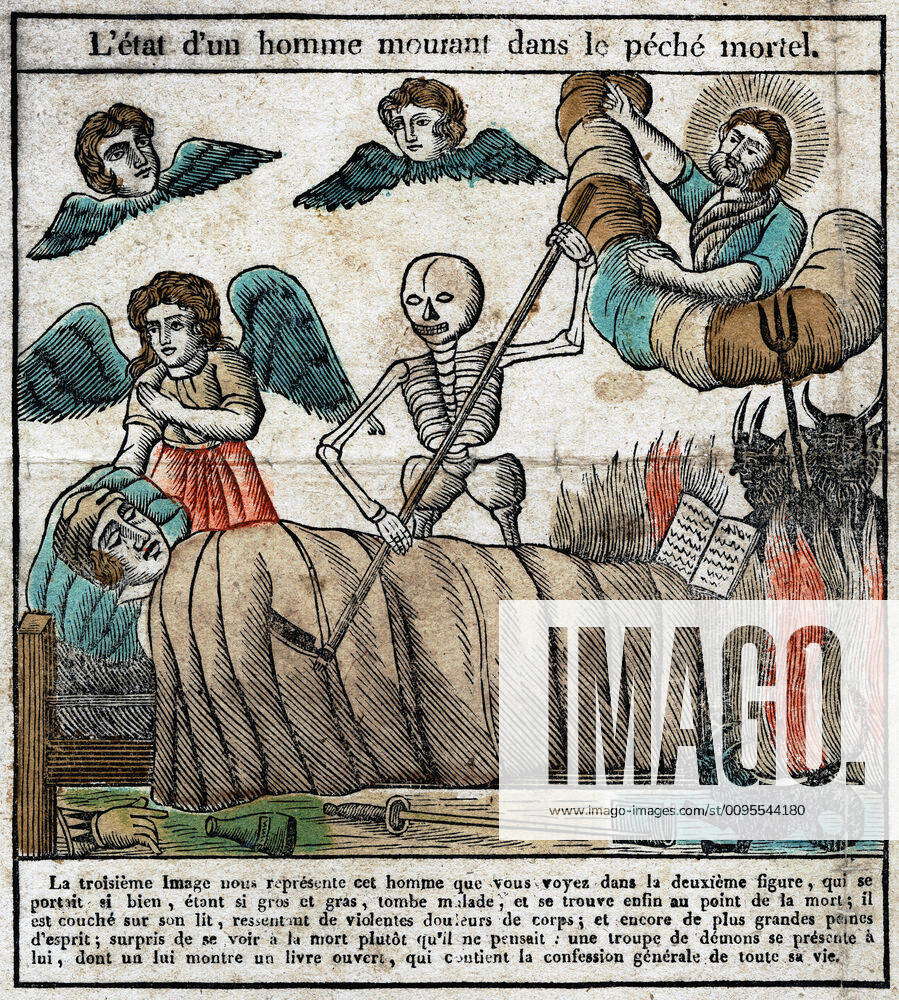This image appears to be an old, faded illustration from a French text titled "Le Tat Dune Homme Murant Danse Le Peche Mortel." The scene is richly detailed: a pale, ill-looking man lies in bed, draped in a light brown sheet and wearing a nightcap. A skeleton holding a sickle or scythe stands over him, the weapon piercing his chest. Surrounding the tableau, two floating heads with blue wings are depicted as angels, while at the bottom right, another angel with wings and a halo is placing a hand gently on the man's head. The background includes a god-like figure with a radiant halo pointing to the sky, his body leant over a color-striped cloud. Two demon-like figures, one clutching a pitchfork, stand menacingly at the foot of the bed beside a book filled with lines of text. Additionally, the illustration includes some French text both at the top and the bottom, along with a watermark in the lower right corner reading, "Imago," followed by the URL www.imago-images.com/st/0095544180.